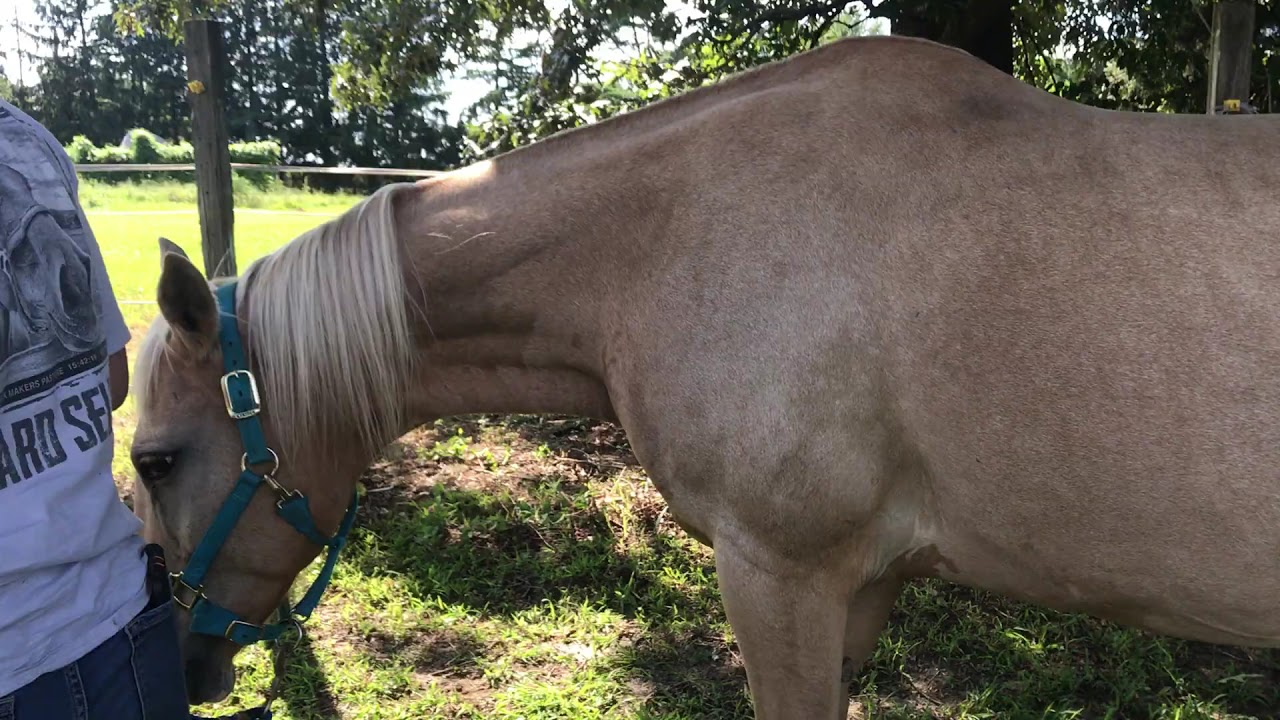The image showcases a tranquil scene featuring a Palomino horse and a person standing together. Dominating the foreground, the horse displays a light tan coat with a thin, blonde mane and wears a turquoise harness around its head and muzzle. The horse's side profile demonstrates a gentle posture with its head lowered, as if engaging curiously with something near its waist. 

On the far left, partially visible, stands a person wearing a white t-shirt adorned with the image of a horse and the words "Hard Sell." Their attire includes dark blue jeans with a noticeable black object tucked into the back pocket. Both horse and human occupy a serene setting beneath the shade of a grove of trees, where light filters through the foliage, creating dappled patterns on the ground.

In the background, there is a brown post without a fence attached, signifying an open and expansive grassy field that extends toward a lush border of green trees. The photograph captures the peaceful interaction between the horse and its likely caretaker against the backdrop of nature’s calm.